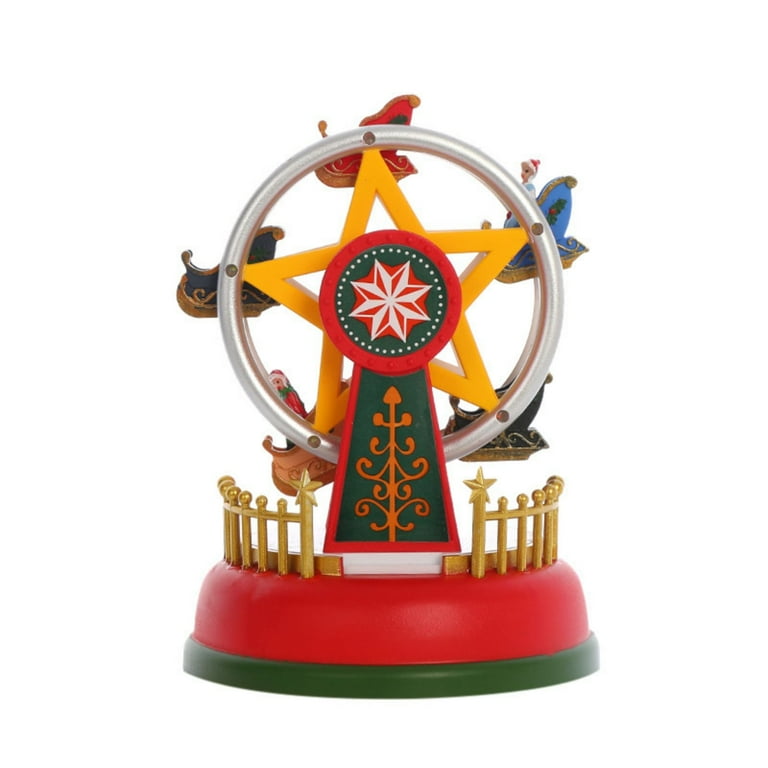A charming miniature ferris wheel is set against a simple white background. The intricate design features a base coated in a lustrous gold hue, topped by a thicker red section. Surrounding the ferris wheel is a light brown fence, with two entrance posts adorned with golden stars. The centerpiece of the ferris wheel is a large, radiant star with a gold exterior and a red circle at its core, which houses a smaller red and white star. The structure expands towards the bottom, supporting five colorful chairs in shades of red, brown, and blue. The overall appearance is delightfully whimsical, making it a captivating little ferris wheel.